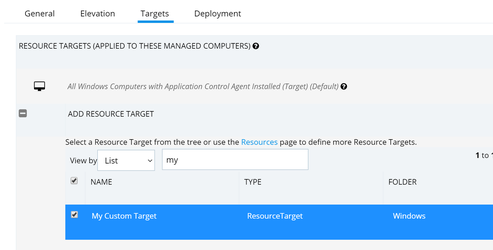This screenshot showcases a section from a Managed Computers page, likely designed for technical support purposes. At the top of the page, there are drop-down menus labeled General, Elevation, Targets, and Deployment, providing navigation options for different categories. Below these menus, a header reads "Resource Targets (Applied to These Managed Computers)," indicating the section’s focus on target management.

The page contains a prompt to "Add Resource Target," allowing users to select or define resource targets via a tree structure or the Resources page. There are two interactive fields: one labeled "View By" with a drop-down menu set to "List" and an adjacent search box containing the placeholder text "My". 

In the main content area, a table is presented with columns named Name, Type, and Folder, the first of which is currently checked. The table lists resource targets, with a highlighted entry in a vivid fluorescent blue labeled "My Custom Target, Resource Target, and Windows," indicating it is selected. The overall design employs a muted color scheme of gray and white with blue highlights to denote selected items.